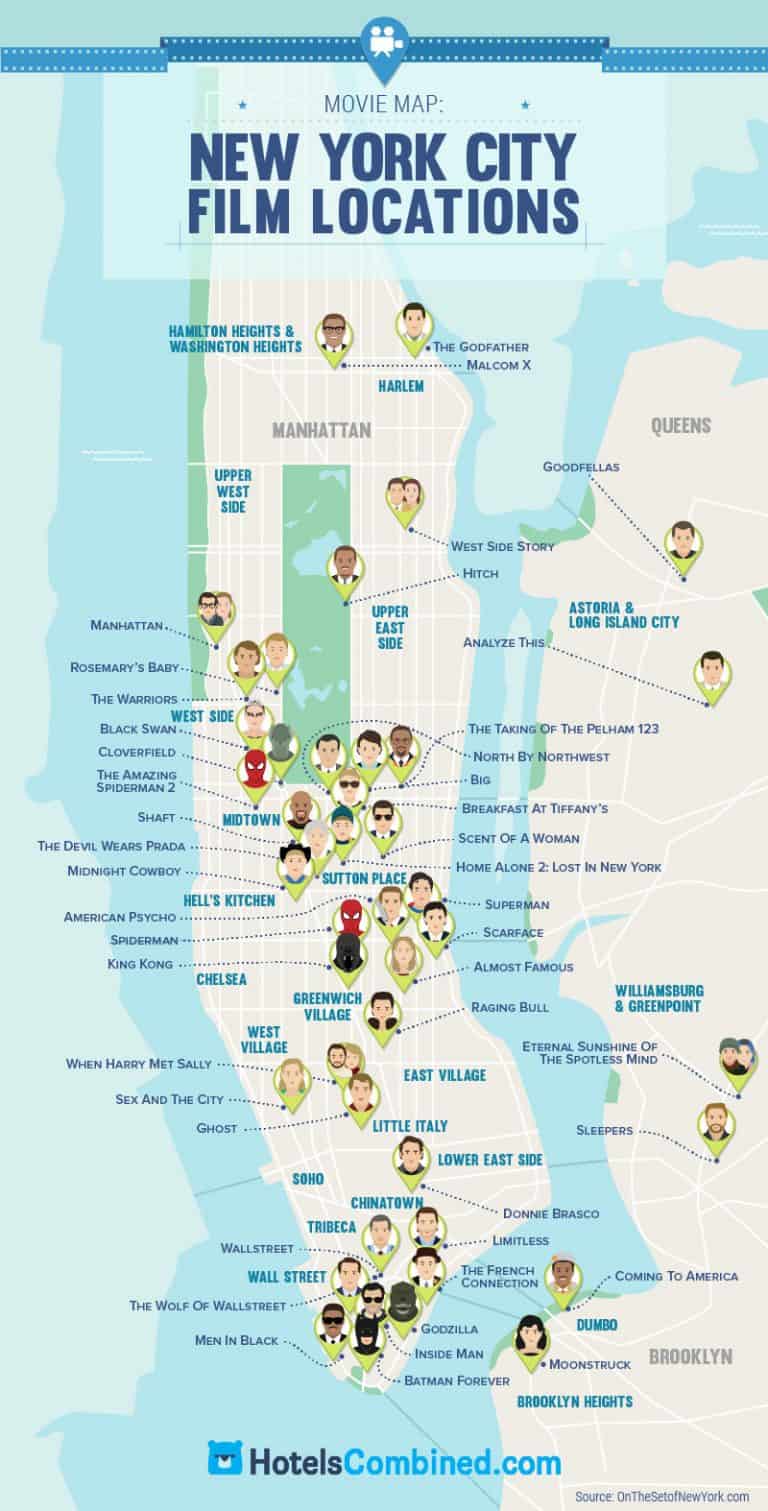The image is a poster entitled "New York City Film Locations" prominently displayed at the top in dark blue text, with an illustrated map of New York City beneath it. The map is marked with several pinpoint icons, each containing cartoon or digital images representing characters or scenes from various films. Notable film titles listed include "The Godfather," "Malcolm X," "Goodfellas," "West Side Story," "The Amazing Spider-Man 2," "Shaft," "Midnight Cowboy," "American Psycho," "Spider-Man," "King Kong," and "Wall Street," among many others. These icons appear throughout different areas of the map, including Manhattan, Queens, and other boroughs, highlighted in a bluish-green color. Towards the center-top of the map, you can see place names like Hamilton Heights and Washington Heights, with various small text labels denoting specific film locations. One notable pinpoint near Midtown features Spider-Man’s face. A zig-zaggy white stripe runs across the top of the poster, adorned with a teardrop-shaped icon at its center. The poster is branded at the bottom with "HotelsCombined.com."